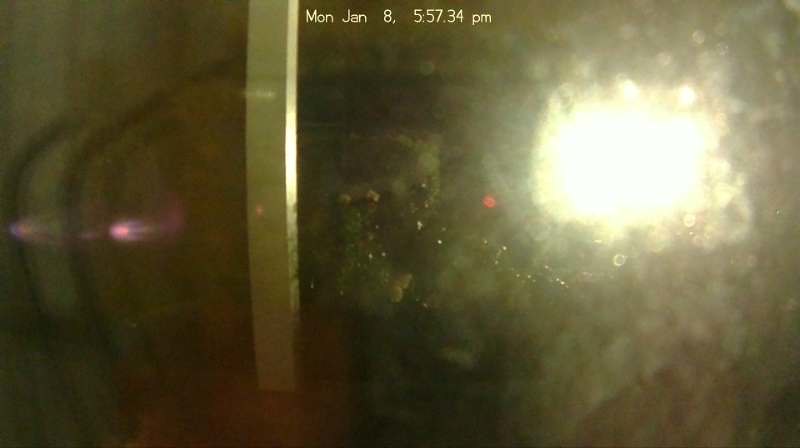Security footage captured on a tablet displays the date and time: Monday, January 8th, at 5:57:34 p.m. The scene is an indoor setting, possibly a parking garage. The right side of the image is blurry due to a dirty camera lens, and there is a single light source on that side. A pillar can be seen in the shot, adding to the garage-like appearance. The bottom floor surface appears to be in poor condition.